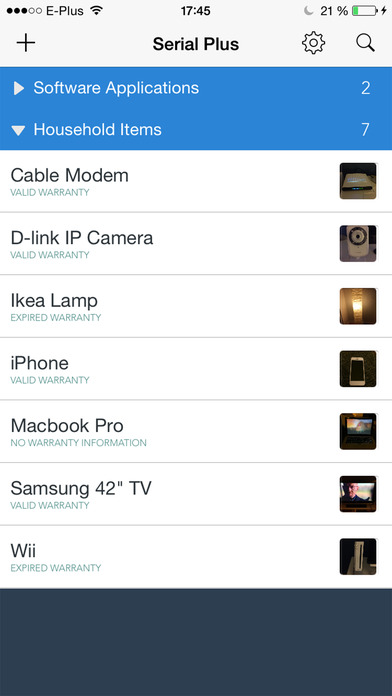This image is a detailed screenshot likely taken from a mobile application managing household items and software. At the very top, there is a header that reads "Serial Plus," accompanied by icons: a plus sign, a gear symbol on the right, and a magnifying glass further to the right. The status bar shows three out of five circles filled, indicating the signal strength, followed by "E-plus," a Wi-Fi symbol, the time displayed as 17:45, a moon icon indicating Do Not Disturb mode, and the battery level at 21%, with a small portion filled in green.

Below the status bar, there are two connected royal blue rectangles labeled "Software Applications" with a downward arrow, and "Household Items." "Software Applications" ends with the number 2, and "Household Items" ends with the number 7, both in white text. 

Scrolling down the list of household items, the entries are: "Cable Modem" marked as "Valid Warranty," followed by "D-Link IP Camera," "Ikea Lamp," "iPhone," "MacBook Pro," "Samsung 42-inch TV," and "Wii."